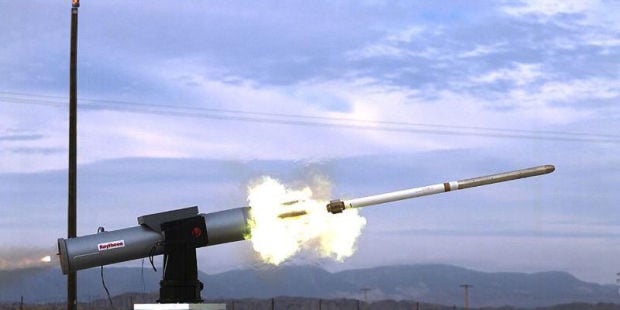This image captures a dramatic outdoor scene, presumably during daylight hours, although the sky is shrouded in dense fog with purple and blue tones, evoking the ambiance of either a cloudy day, sunrise, or sunset. The focal point of the photograph is a powerful moment of a artillery cannon firing a rocket or small missile. The launcher itself is a gray rocket grenade launcher housed in a black mechanical arm or cradle, attached to a metal plate. Various details such as multiple cables running off the sides, a white label with unreadable red writing, and a red light are visible on the launcher. 

As the rocket emerges from the barrel, an impressive burst of blurred white and yellow flames is visible, resembling a rapid and intense fire. The rocket itself features a white rear, a dark brown tip, and a body colored with shades of brass and gray. The rocket also has small steering fins at the end. 

In the backdrop, you can make out a vague outline of mountains shrouded in thick fog. Additionally, there is a large pole on the left side of the image extending from the base to the top, likely a power line, with visible lines stretching out to the right. Further adding to the dynamism of the scene, another burst of light is discernible in the distant background, suggesting a second launcher might have been fired.